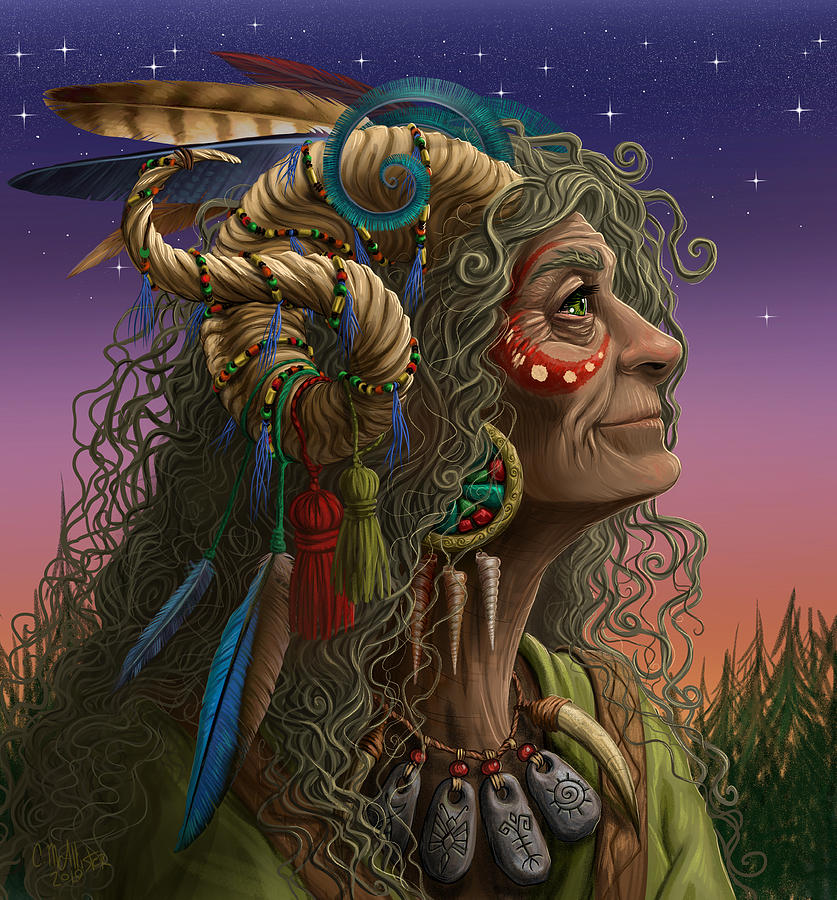This incredibly detailed illustration portrays an elderly Native American woman with weathered, leathered skin marked by fine lines and wrinkles. Her profile reveals bushy gray eyebrows and piercing bright blue eyes that gaze forward. Her face is adorned with a prominent red crescent moon-shaped paint featuring white and golden dots below her eye. She wears an intricate and ornate headdress woven with an array of red, blue, and brown feathers interspersed with red tassels, and a unique blue feather curling gracefully like a peacock's tail.

Her wild, long, gray and gold straw-like hair spills out from beneath the headdress, adding to her mystical appearance. Between her horns, the headdress sits prominently. Large woven earrings with turquoise and red coral, embellished with metal pieces in the shape of shells, dangle from her ears. Around her neck rests a necklace adorned with four metal silver objects, each inscribed with Native symbols, and additional stones embedded in it, some appearing to be ornately carved.

She is depicted wearing a green blouse-like outfit. The sky in the background transitions dramatically from a deep purple at the top to shades of pink and orange closer to the horizon, filled with twinkling white stars. A few trees stand tall on the right side of the image, adding context to the scene. The overall effect is colorful yet dark, exuding a mystic aura.